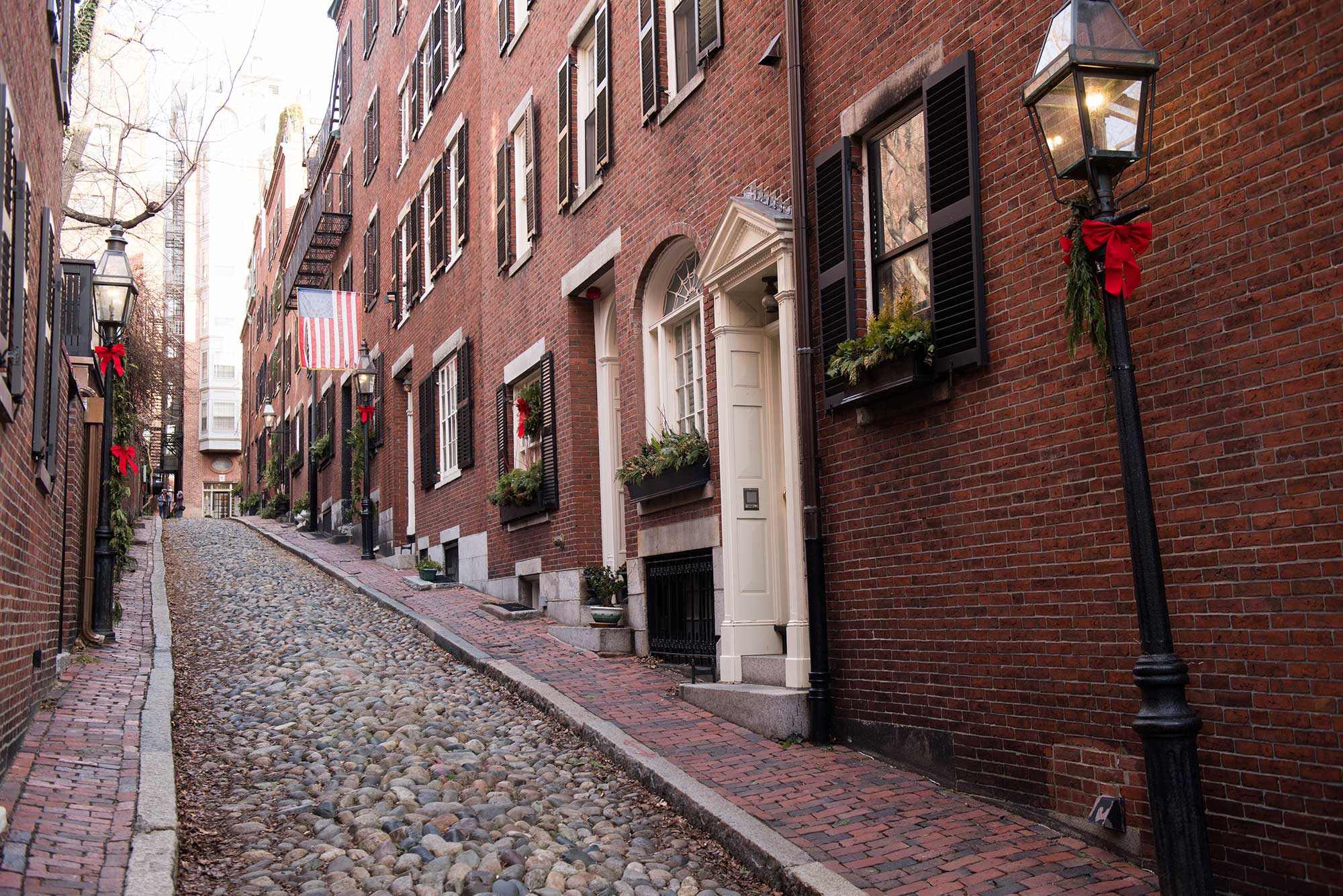This photograph captures a charming, historic cobblestone alleyway framed by tall, red-brick rowhouses evocative of colonial-style architecture. The narrow street, flanked by brick sidewalks with skinny concrete curbs, winds gently upwards. Decorated for the holiday season, the black metal street lamps lining the alley are adorned with red ribbon bows and green garlands. Window boxes bursting with greenery add to the festive atmosphere, while the doors, mostly painted white, contrast against the reddish-brown brick façades. The buildings are likely four stories high, although some descriptions suggest they may stretch up to five stories. Black shutters accentuate the windows, and an American flag is prominently displayed from a building on the right side. The alley's slight incline leads the eye upwards, and the bright, whitish sky hints at an early morning. In the background, a taller structure, possibly a church steeple or school tower, adds to the quaint, picturesque scene that resembles historic streets found in cities like Philadelphia or Boston.